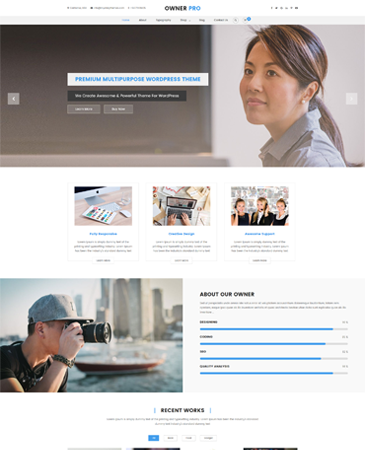The image showcases the homepage of a website named "OwnerPro." The website's name is prominently displayed at the upper center of the page. Directly below the OwnerPro title is a center-aligned navigation menu consisting of six items. Beneath the menu is a full-width banner featuring an image of a woman with brownish hair tied back in a ponytail. She is wearing a gray shirt and has her body turned towards the left of the image, although her face is angled towards the bottom left. Within the banner, to the left of the woman, is a white box containing the text "Premium Multipurpose WordPress Theme." Below the banner, there is a white section that houses three distinct boxes, each containing a different picture.